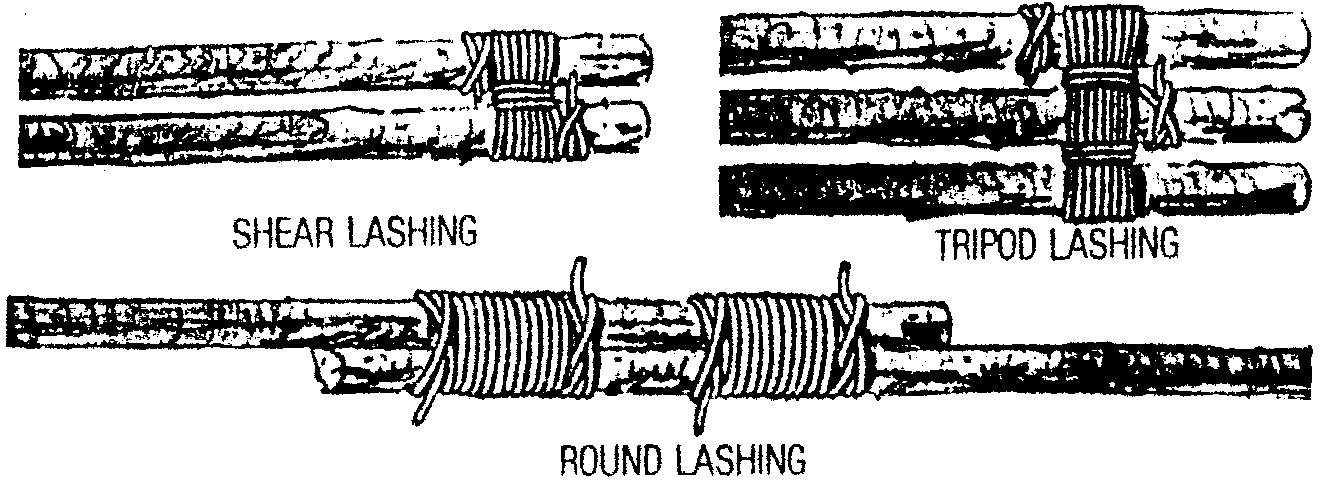The image showcases three detailed sketches of traditional lashing techniques, frequently used in tent-making or similar structures, possibly by American Indians or indigenous communities. In the top left corner, the sketch labeled "Sheer Lashing" illustrates two horizontal sticks bound together at the right side with a heavy string. The top right corner features "Tripod Lashing," showing three sticks tied horizontally in a similar manner. At the bottom, "Round Lashing" depicts two sticks overlapped and secured at two points, somewhat off-center, resembling an extended telescope. The image is rendered in black, white, and gray, giving it a worn, photocopied appearance, likely intended for educational purposes.